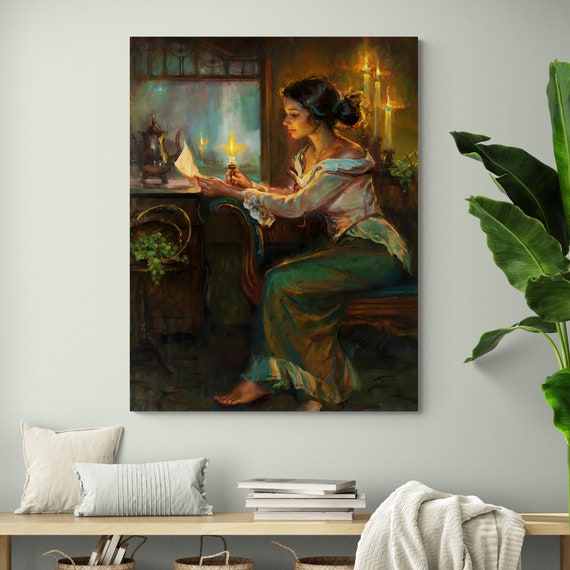In this image, a painting hangs prominently on a light blue wall adorned with a picture of a woman reading a letter. The woman, with black hair in a ponytail and dressed in a white off-shoulder shirt and a long, green skirt with light green frills and black dots, holds a piece of paper in her left hand and a pen in her right, suggesting she's writing. She sits on a blue and wooden chair, facing left. There's a lantern in front of her lighting a mirror as three candles burn behind her in an antique setting. Partially visible in the room is a large green leafy plant with two-foot-long leaves, along with a wooden shelf below the painting. On the shelf, there are two pillows—a square one propped against the wall and a tube-shaped one lying down—beside a stack of four or five books. Draped over the edge of the shelf is a fuzzy blue bathrobe. Beneath the shelf, three wooden buckets add a rustic touch to this modern living space.